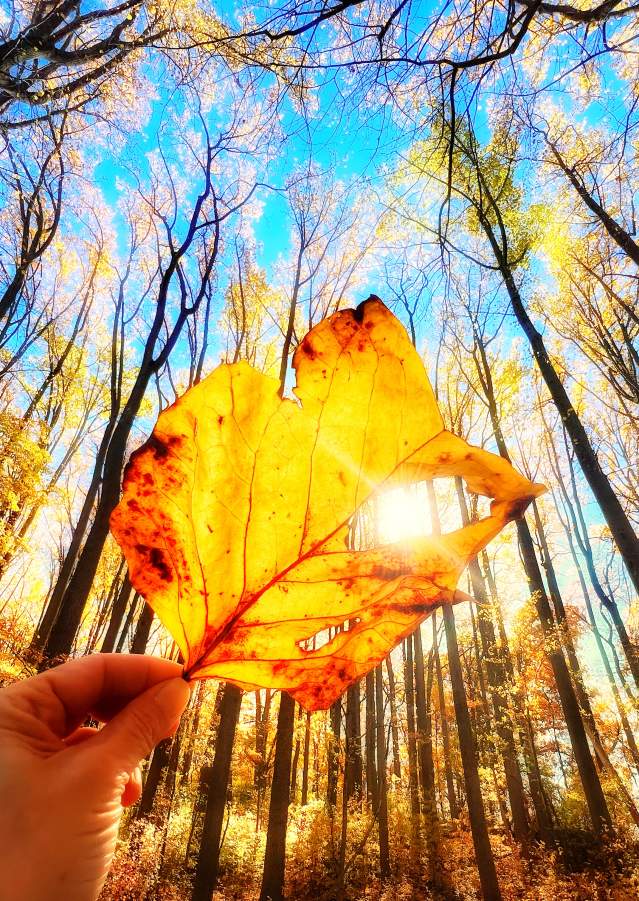In a sunlit forest, a person holds up a leaf by its stem in their left hand. The leaf, tinged with warm autumn colors of orange and yellowish-orange, is central in the image. The scene is bathed in natural light from a clear blue sky, highlighting a small, off-center hole in the leaf through which the sun shines brightly. The hand holding the leaf is positioned in the bottom left corner of the frame, offering a creative visual where the sun piercing through the leaf adds an intriguing focal point. Surrounding the leaf, abundant green foliage, tree bark brown trunks, and scattered yellow hues paint a picturesque daytime forest backdrop.